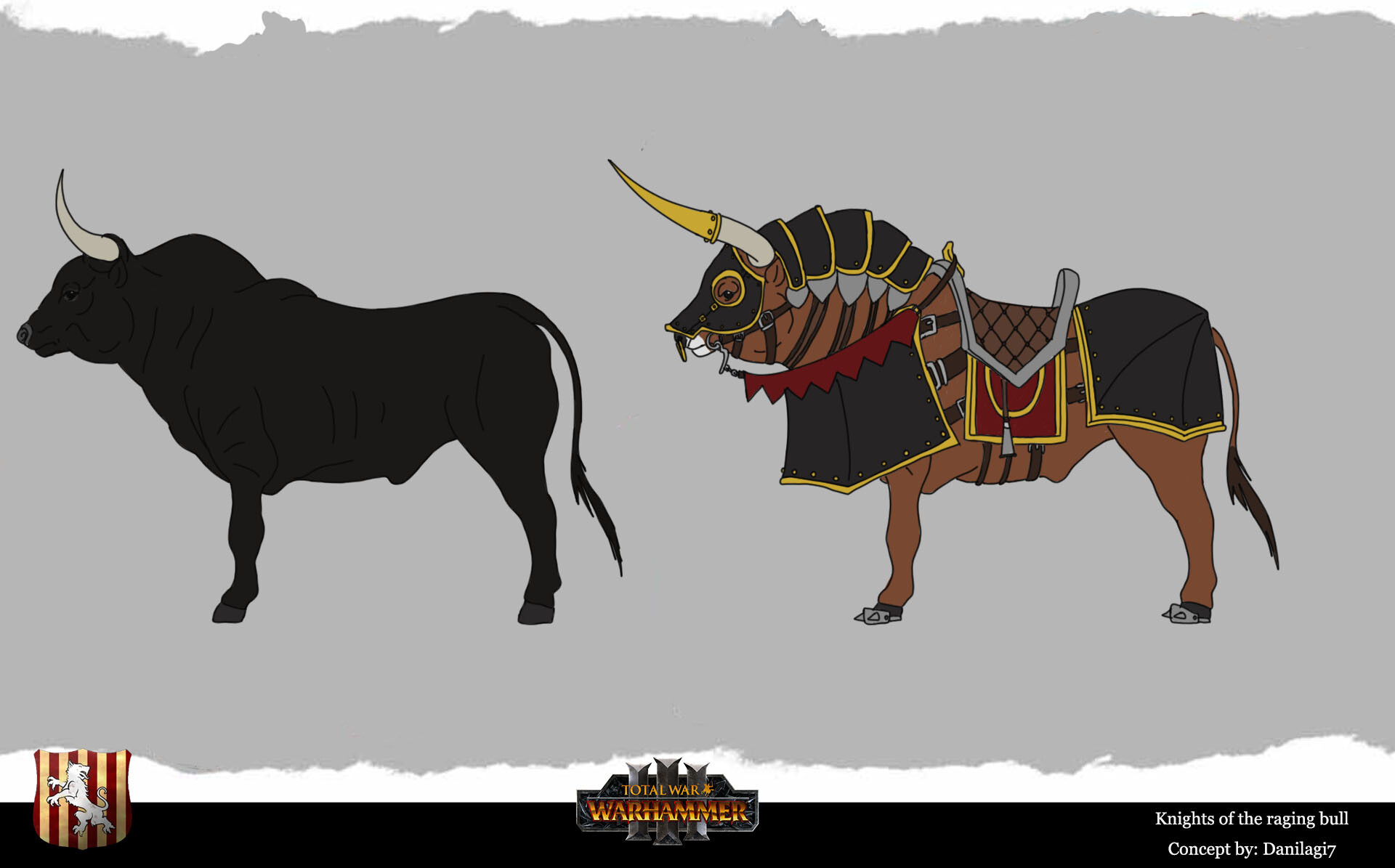This detailed illustration prominently displays two bulls set against a simple gray background with rough edges at the top and bottom. The bull on the left is a black silhouette with strong, cream-colored curved horns and a long tail, facing left in profile. The bull on the right contrasts with a light brown hue, embellished with extensive armor: a metal cap screws into its long horns, scaled segmented armor covers its shoulders, and additional armor guards its face, neck, chest, and rear. This armored bull also features a burgundy cloth banner and a saddle for riding. Both bulls are part of a concept titled "Knights of the Raging Bull," credited to DanellaGI7, with the title "Total War Warhammer" appearing at the bottom right of the image.